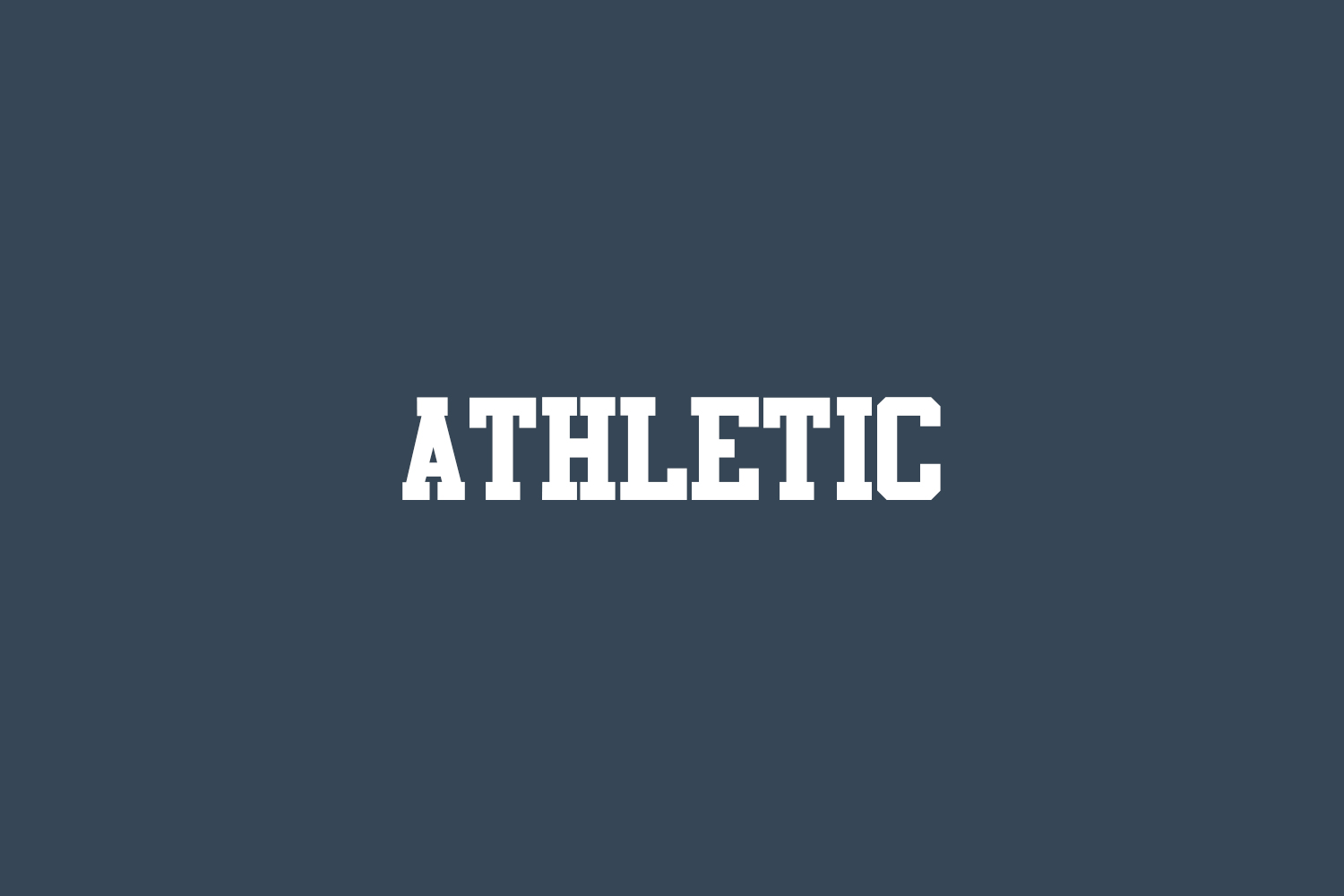The image is a simple, horizontal rectangular design featuring the word "ATHLETIC" prominently centered both vertically and horizontally. The background is a solid, uniform color that could be described as either a dark charcoal gray or a subtle black. The text is written in all capital, block letters, making it easily readable and visually striking against the dark background. The font size appears to be around 28 points, though the exact typeface is unspecified. The image is clean and minimalist, with no additional pictures, words, or website references—just the single word "ATHLETIC" in the middle, standing out clearly and uniformly against the solid background.